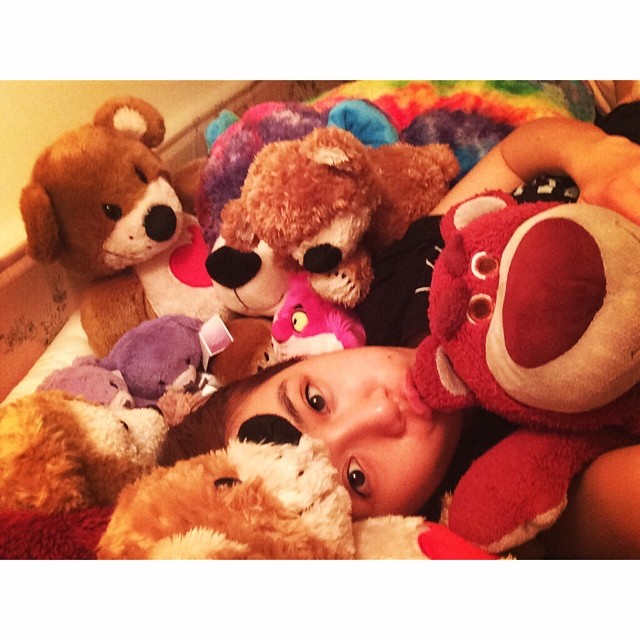In the center of this color photograph, taken inside what appears to be a child's room, a young person lies on a bed, surrounded by a vibrant assortment of stuffed teddy bears. The person, possibly a teenager with dark brown hair pulled back and expressive dark brown eyes, is gazing up, making direct eye contact with the viewer. They are wearing a dark shirt and possess a tan complexion.

Piled around them on the bed are teddy bears of various colors and types. Notably, the large pink bear with a dark pink nose from Toy Story 3 occupies the right side of the image. This bear, known for its role as the mean bear in the movie, is closely embraced by the person, who is tenderly kissing its ear.

Among the stuffed animals, there is a brown bear at the top with a red heart on its chest, a purple bear, a bright pink bear with yellow eyes, and a rainbow-colored stuffed creature featuring shades of orange, yellow, green, and dark purple. The cozy, whimsical scene shows the individual affectionately clutching the Toy Story bear, their hand wrapped around it, creating a heartwarming snapshot of youthful adoration amid a plush menagerie.